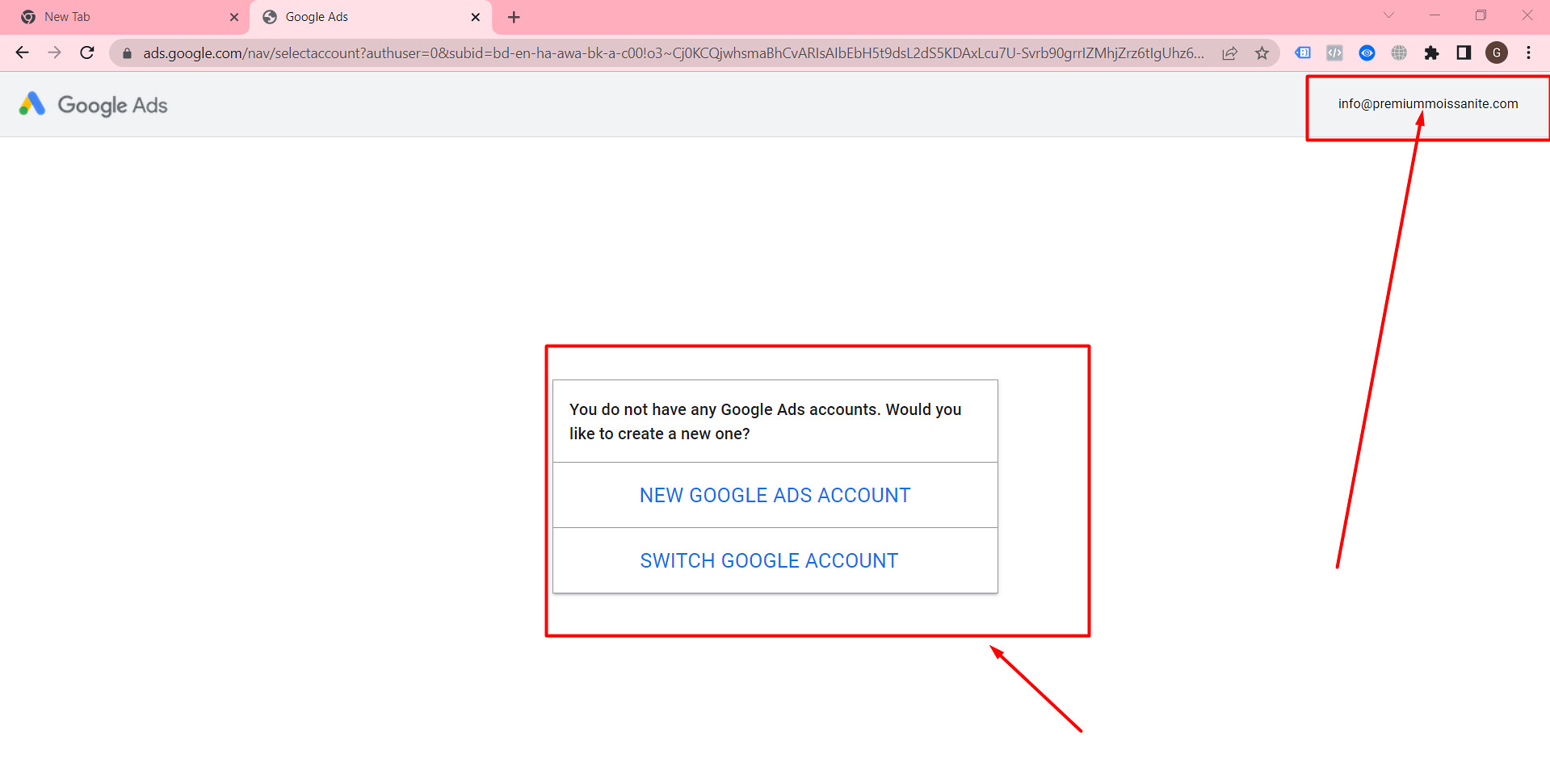This screenshot captures a web page displayed on a Google Chrome browser, specifically highlighting the Google Ads interface. The browser's top ribbon bar, shaded in pink, clearly marks the active tab as "New Tab" on the left side. Adjacent to it, a second tab is open and labeled "Google Ads," indicating the page currently in focus.

In the upper right section of the browser, you can see the standard navigational buttons, including left and right arrows, a reload button, and the omnibox displaying a detailed URL filled with numbers and text parameters indicative of a specific Google Ads page. Various Google Chrome extensions are also visible on the right side of the omnibox, alongside a Google account avatar and the iconic three vertical dots representing additional settings.

Lower down on the page, a gray header bar prominently features the Google Ads logo and "Google Ads" text. To the right within this header, there's an email ID associated with the logged-in account. Centrally located within the main content area of the page, a red-colored dialog box stands out, drawing attention with the message, "You do not have any Google Ads account. Would you like to create one?" The top right section, including the Gmail bar, is also marked with arrows and highlighted, presumably to guide the user’s attention to specific interactive elements related to account setup or navigation.

This detailed description encapsulates the screenshot's core visual and contextual elements, effectively guiding the viewer through the various components of the Google Chrome interface and the Google Ads web page in question.